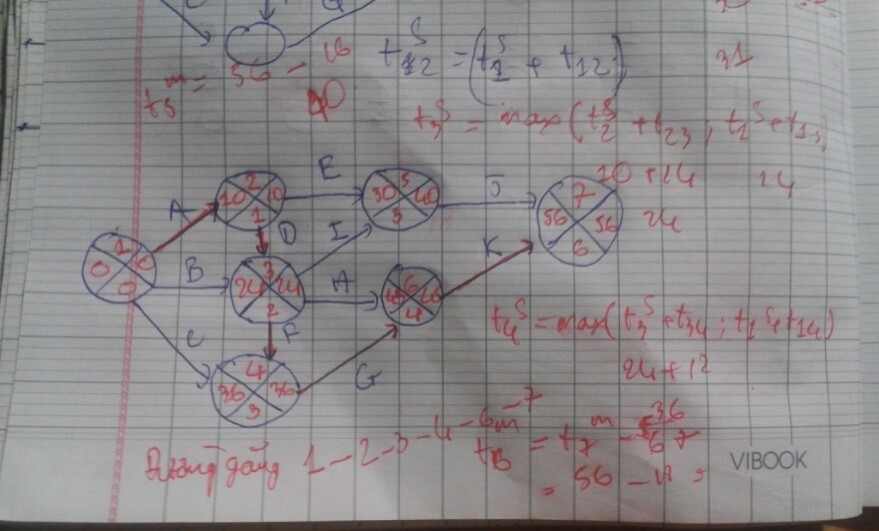This photograph captures a notebook page densely packed with handwritten mathematical formulas and equations, meticulously inscribed in blue and red ink. Prominently featured on the page, there is a matrix-like arrangement of interconnected circles, each subdivided into four quadrants. Within each quadrant, numbers are neatly written, such as "0, 0, 2, 0" in one circle and "10, 2, 10, 1" in another. These numbers suggest some form of numerical or algebraic analysis, potentially involving the calculation of maximum and minimum values. The detailed and colorful annotation reflects a comprehensive attempt to solve or illustrate complex mathematical problems.